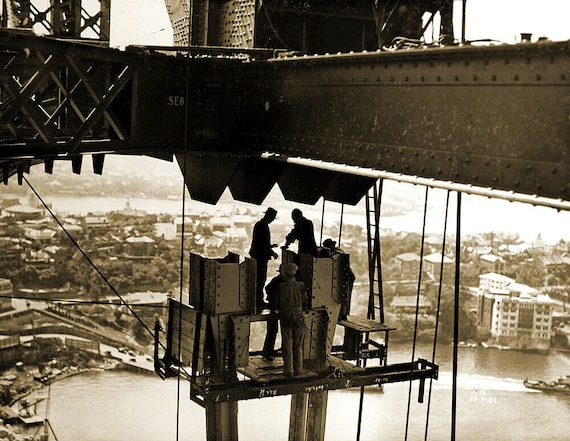This sepia-toned vintage photograph, dated September 25, 1930, captures a group of construction workers standing on steel girders and scaffolding, high above a sprawling cityscape, likely during the erection of a bridge or high-rise building. The men are each focused on different tasks among a web of riveted metal panels and I-beams, silhouetted against the sky. The photograph is taken from an elevated vantage point and slightly distanced, providing a sweeping view of the bustling city below. In the background, a vast body of water, possibly a river or lake, snakes through the urban landscape, dotted with boats and flanked by clusters of buildings and tree-dotted neighborhoods. The depth of field renders the distant cityscape and waterways slightly out of focus, emphasizing the height and precariousness of the workers' environment. One notable detail is a worker in shadow donning a top hat, adding a unique period charm to this industrial scene set against the sepia-toned backdrop of a bygone era.